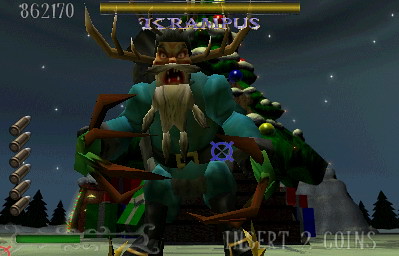This image is a detailed screenshot from an arcade game. The game's user interface prominently features a player health bar located in the bottom left corner of the screen. Dominating the center of the image is a menacing, fantasy character that appears to be an old man with a long beard and large deer antlers protruding from the sides of his head. This character's name seems to be "Krampus," aligning with the theme of an evil Christmas demon. In the background, there's a Christmas tree, adding to the holiday-themed atmosphere of the game.

Additionally, the interface shows six bullet icons along the left side of the screen, indicating the player's ammunition count, and a yellow score and health bar up top. The bottom right corner displays the text "INSERT 2 COINS," confirming that this is indeed an arcade game, as inserting coins is a common feature for such games, unlike typical console or PC games.